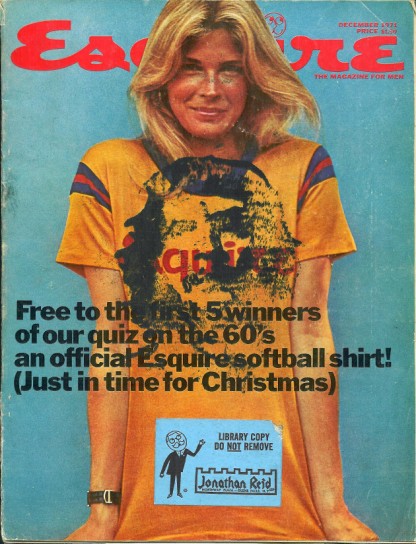This is a detailed photograph of an Esquire magazine cover featuring a blonde woman wearing an orange shirt. She stands with her arms at her sides and a slight smile on her face, without showing teeth. The orange shirt prominently displays the Esquire logo in red text in the middle, complemented by additional text at the top of the cover also reading "Esquire" in red. The black bold text across the cover highlights a special offer: "Free to the first five winners of our quiz on the 60s - an official Esquire softball shirt just in time for Christmas." Additionally, there is a white sticker affixed to the bottom of the shirt with the following text in all capital letters: "LIBRARY COPY DO NOT REMOVE." The word "NOT" is underlined, and beneath this text, the name "Jonathan Reed" appears in smaller print. Adjacent to the name is a graphic resembling a Monopoly-style old man icon. The woman also wears a watch strap on her right wrist. The color scheme includes teal, red, orange, navy blue, white, and black, suggesting a digitally created or software-enhanced print.